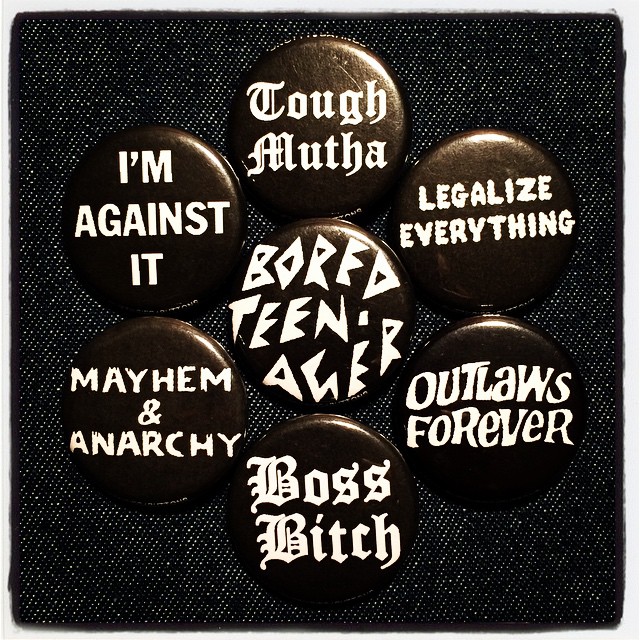The image displays a square swatch of black denim fabric with a thin white border along its edges. The fabric has a peppered appearance, interspersed with tiny white dots, and features stitching around the perimeter. At the center and around the swatch are seven circular buttons, each adorned with distinct white text in various fonts. The central button prominently reads "Bored Teenager" in bold, blocky lettering. Surrounding it in a clockwise fashion are: a top button at the 12 o'clock position with gothic-style text saying "Tough Mutha," followed by "Legalize Everything" in cloudy, stylized print, "Outlaws Forever," "Boss Bitch" in another gothic style at the 6 o'clock position, "Mayhem and Anarchy," and finally "I'm Against It" in bold, clear letters.